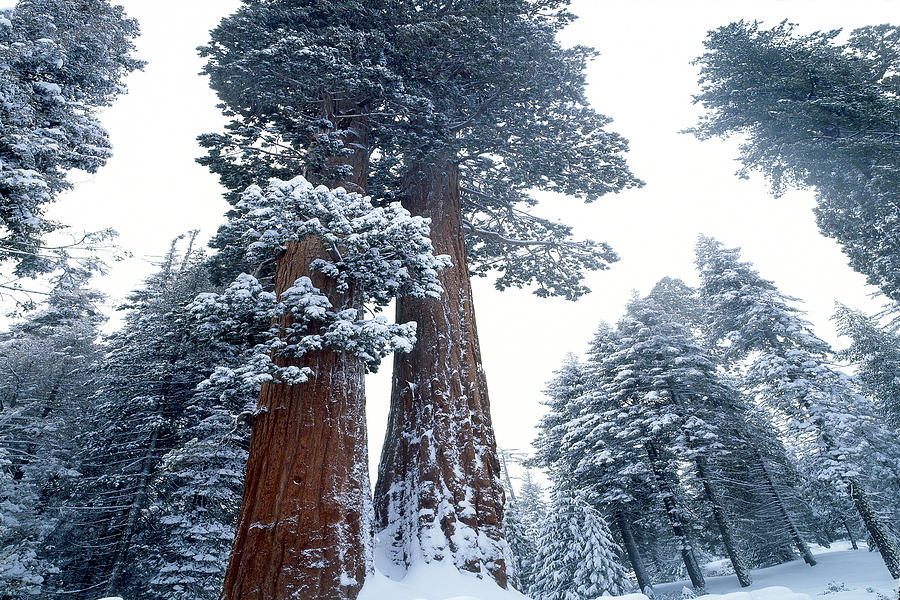The photograph depicts a serene winter forest scene on a bright, cloudy day. Dominating the center of the image are two exceptionally tall trees with thick, dark brown trunks, extending upward from the bottom of the frame. These central trees are unique in that their trunks are more visible, with just a light dusting of snow near the base. At the tops of these trees, a mix of mint green foliage and white snow creates a striking contrast. Flanking these two central trees are various evergreen pine trees covered heavily in snow, with minimal trunk visibility. The ground, especially on the right-hand side of the image, is blanketed in several inches of snow, adding to the wintery atmosphere. Overall, the interplay of snow-covered branches and the distinct structure of the two prominent trees adds a rich textural depth to the forest scene.